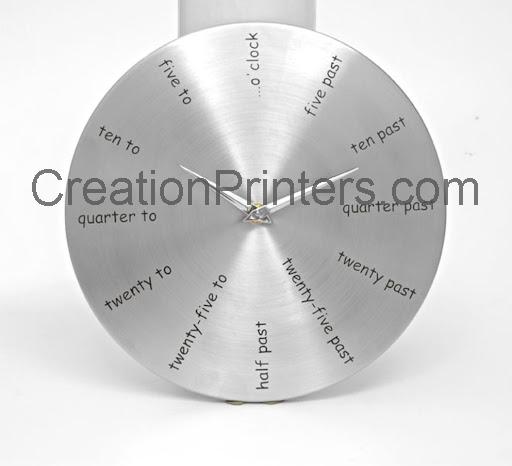In the center of a light gray background, a striking silver metallic disc serves as a unique clock, prominently displaying the text "creationprinters.com" across its middle. This clock, attached to a vertical metal bar, features elegant silver hands. The smaller hand is positioned near 10 to, while the larger hand hovers slightly below 10 past. Around the edge of the disc, black numerals mark time intervals: the top left shows 5 to, the top middle says o'clock, the upper right indicates 5 past, further to the right 10 past, quarter past, 20 past at the bottom right, 25 past, half past, 25 to, 22, quarter to, 10 to, and completing the circle at 5 to. The clean, metallic design casts a subtle shadow, enhancing its dynamics against the contrasting white background. The overall composition is minimalist yet intricate, blending function with aesthetic appeal.